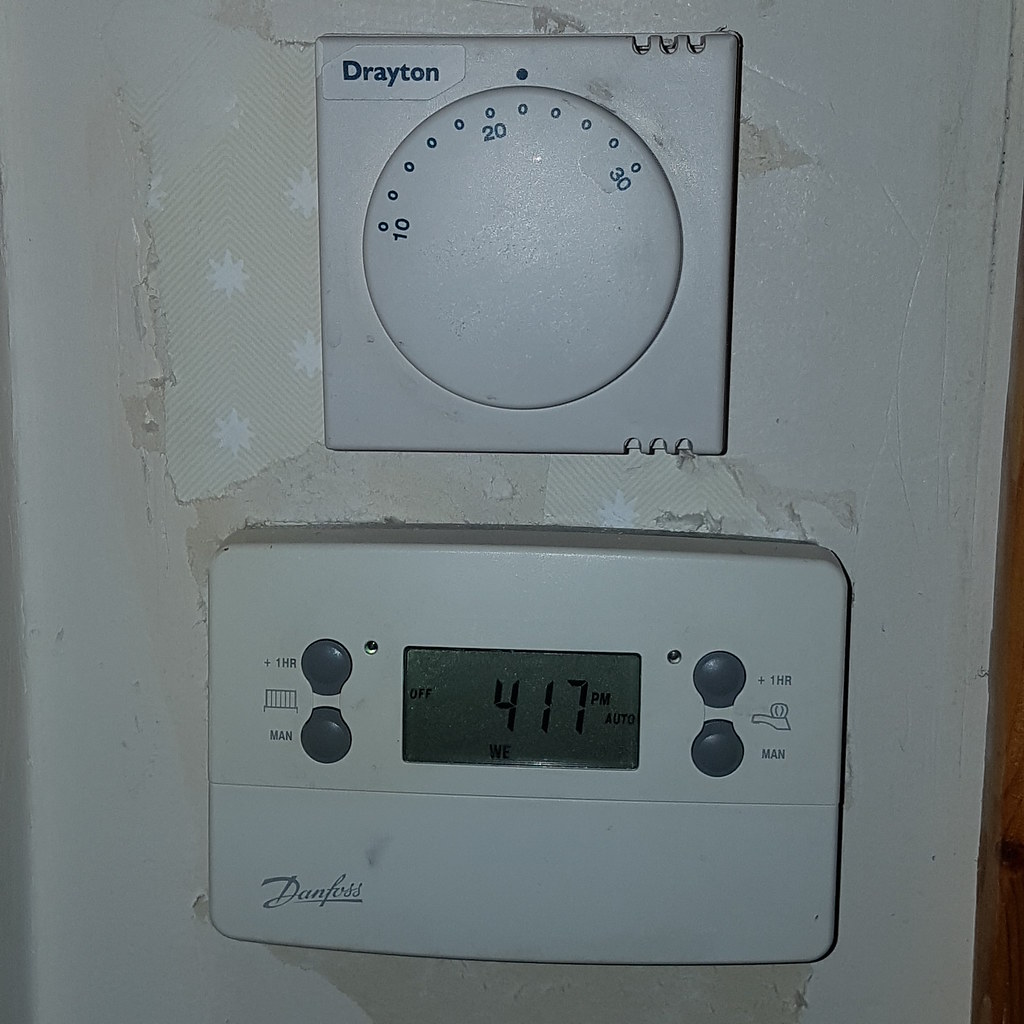This image shows a detailed view of a Danfoss climate control thermostat mounted on a white wall. The device displays the time 4:17 PM and is set to automatic mode, indicated by "AUTO" on the right side of the screen. The current day appears to be Wednesday ("WE"), and the system status is "OFF." 

Above the main display, there is a smaller temperature control screen showing 22 degrees Celsius, which is approximately in the 70s Fahrenheit, typical for a controlled indoor environment. The thermostat has four buttons on each side: the left side has a "+1 HR" button and a button marked "MAN" for manual mode with distinct symbols resembling a mini fence and a faucet. Similarly, the right side also has "+1 HR" and "MAN" buttons with different icons.

The wall behind the thermostat is white but shows signs of damage and repair attempts. The wallpaper has small star patterns, and there are visible patches where white paper has been applied to cover peeling sections.

The brand "Drayton" is visible at the top of the thermostat, and the circular temperature dial ranges from 10 to 30 degrees Celsius, with markings in increments of 2 degrees.